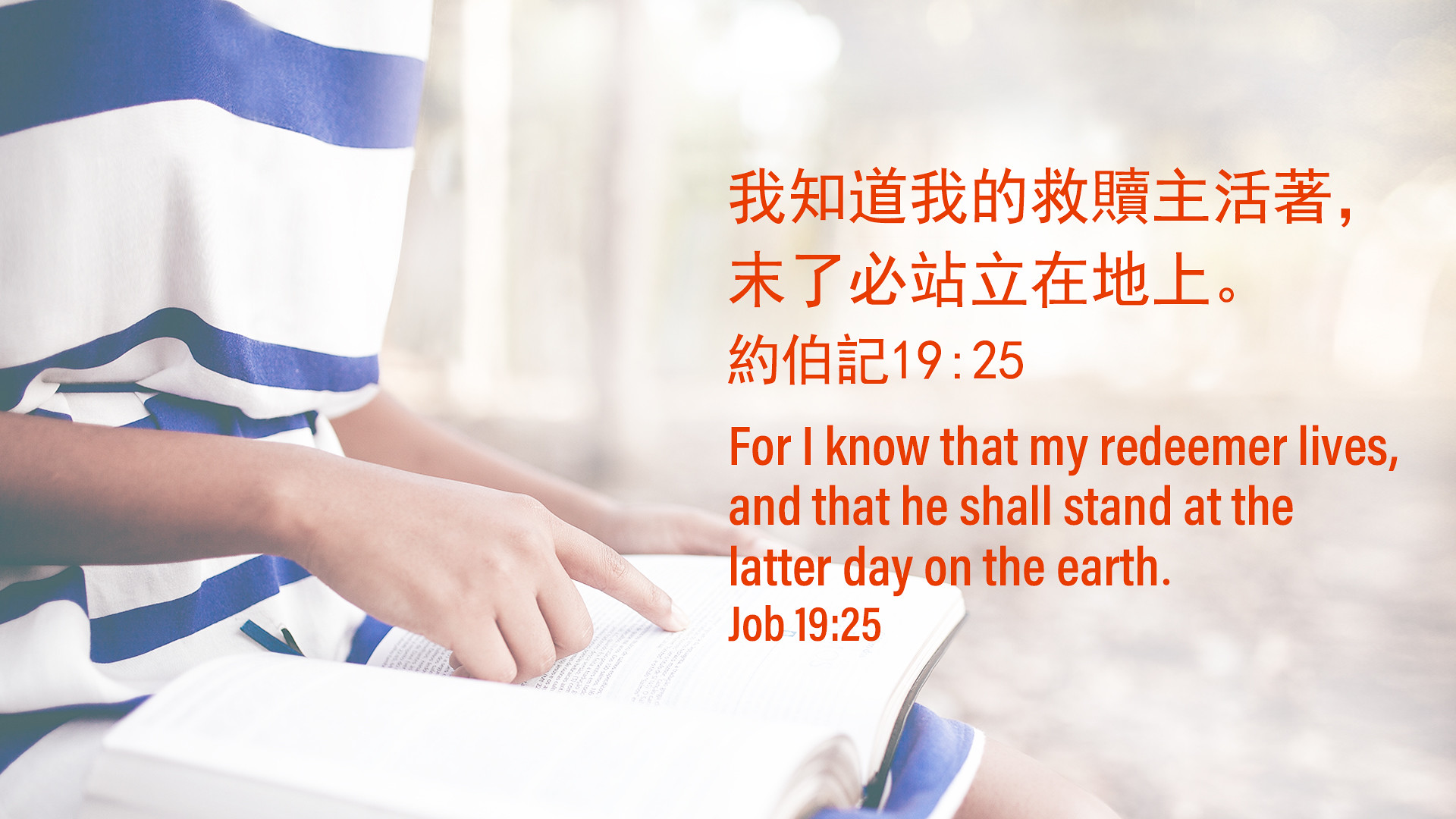The poster, shaped and sized like a large high-definition television, features an outdoor scene that stretches wider than it is tall. On the left-hand side, a young person, possibly a child or teenager, is seated with an open book, likely a Bible, resting on their lap. Their fingers trace the words on the page attentively. Dressed in a blue and white striped shirt, the individual’s face is not visible, focusing attention on the act of reading. The colorful setting includes various shades of blue, white, red, tan, and brown, suggesting it was taken during the daytime.

Adjacent to this scene on the right side of the poster is an inscription comprising two quotes. The first quote is in a language that appears to be Japanese or Chinese. Below it, clearly written in English, is a passage from the Bible: "For I know that my Redeemer lives, and that He shall stand at the latter day upon the earth. Job 19:25." The English text is highlighted in red letters, providing a striking contrast to the soft background, which remains slightly blurred.